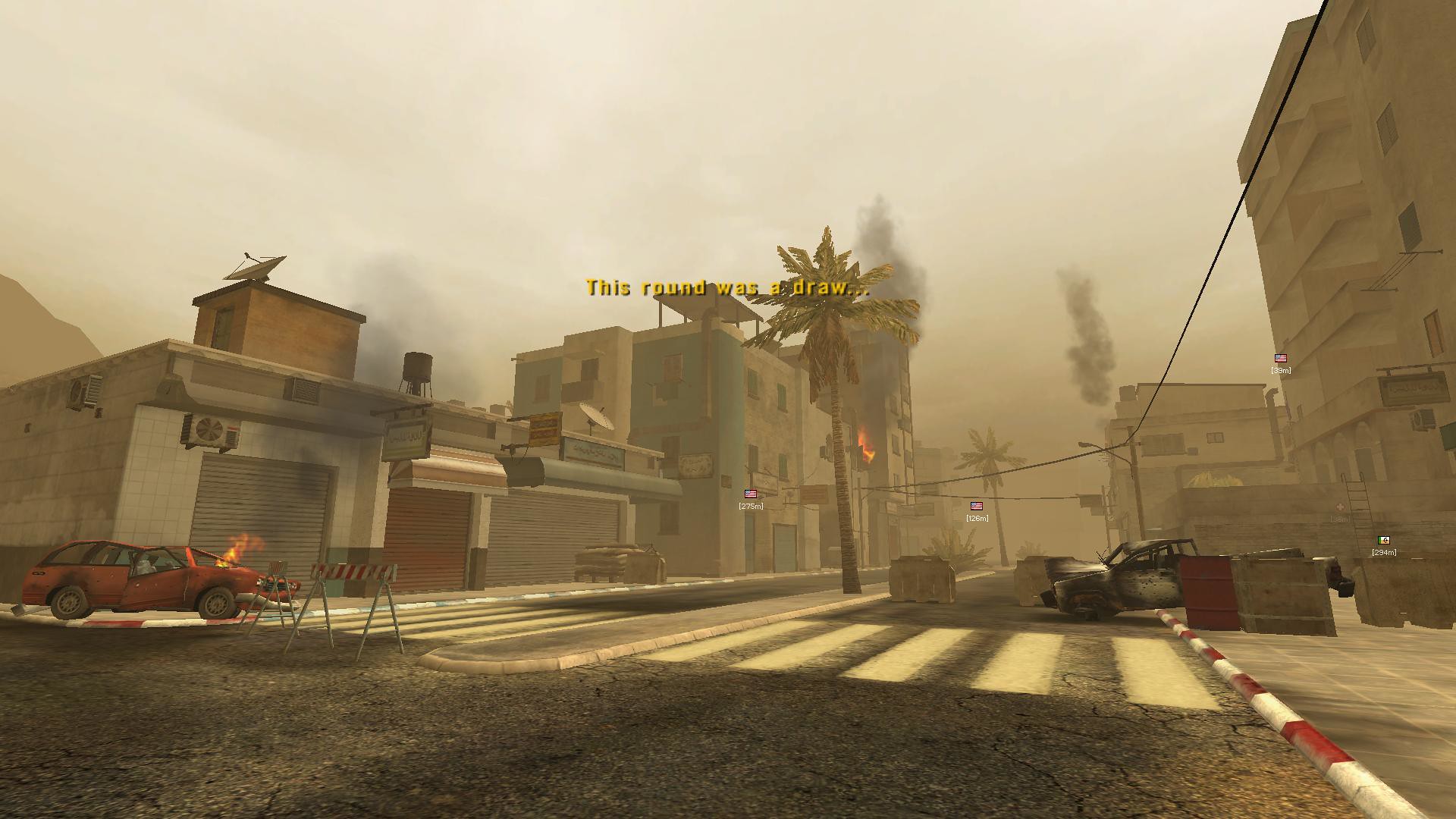In this rectangular, horizontally-oriented scene from a video game, we are presented with a dramatic and chaotic urban setting. The sky is dark and overcast, casting a brooding atmosphere over the scene. A street runs diagonally from the lower left to the upper right of the image, cutting through the center of the turmoil. On the left side of the street, several one-story and three-story buildings stand in a row, suggesting a mix of residential and commercial purposes. The right side features taller apartment buildings.

Adding to the sense of disarray, there is a red station wagon on the left side of the street, its engine engulfed in flames. Nearby, a dark-colored pickup truck appears to have crashed, with its two front wheels suspended over the street and its rear end perched precariously on the sidewalk. Scattered palm trees line the scene, indicating a warm climate despite the stormy sky above. The overall mood conveys a tense moment frozen in the midst of calamity.